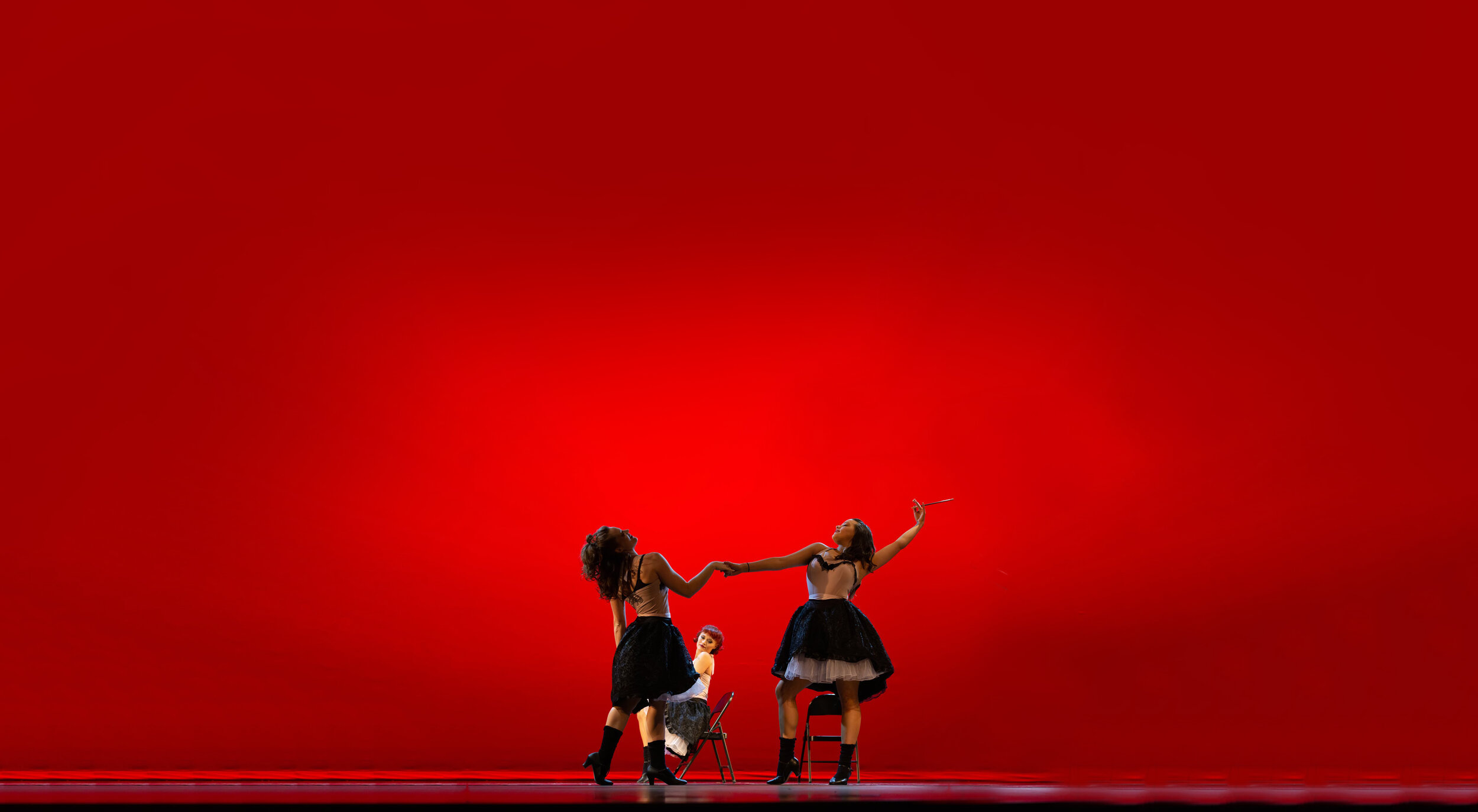In this evocative image, set against a vibrant red background that brightens at the center and fades into shadowy crimson at the edges, three women perform a mesmerizing dance on a stage. The two women in the foreground are adorned in striking outfits consisting of black skirts with tulle that puff out just above their knees, paired with pink and black bustiers and black boots that reach up to their calves. One woman's arm is gracefully raised, with her body leaning slightly back, while the other woman, holding her hand, stretches her arm downward. Their dark hair flows as they move, adding to their dynamic presence on stage. Behind them, partially obscured, sits a third woman dressed in a white tank top and a black skirt. She has medium brown hair and appears to be Caucasian. The stage's floor is likely black, and two black chairs are faintly visible. The interplay of light and shadow, combined with the dancers' expressive poses, creates a captivating visual narrative.